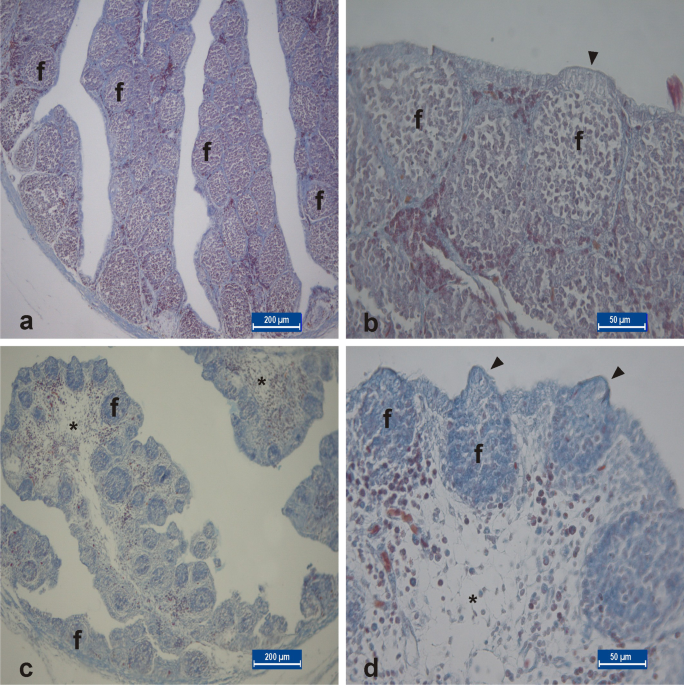The image is set against a plain white background and is divided into four equal-sized photographs, each measuring about two inches by two inches. The photographs are arranged in a grid with two on top and two on the bottom, separated by white borders. The photographs are labeled A (top left), B (top right), C (bottom left), and D (bottom right) in their lower left-hand corners. In their lower right-hand corners, small blue rectangles display white text indicating magnification or other relevant details: A says "200 UPM," B says "50 UPM," C says "200 UM or PM," and D says "50 PM."

All photographs appear to be microscope slides, each predominantly featuring shades of purple and gray. The first image (A) shows a purple-toned background with the letter "F" crossing it and white streaks descending that might resemble blood vessels. The second image (B) is a close-up of image A, highlighting more details with gray and purple tones and featuring a ridge line indicated by an arrow.

The third image (C), labeled in the lower left, zooms further into the gray areas of the previous images, displaying larger white-vein structures and marked with an asterisk. The final image (D), located in the bottom right, introduces a bluish tone to the overall gray and white palette. Here, raised areas are marked, which could resemble tips or points, and the observer noted whitish, possibly nail-like elements protruding from the gray mass.

Although the exact subject remains unclear, the detailed structures and varied labeling suggest a scientific or medical context, possibly related to histology or pathology.